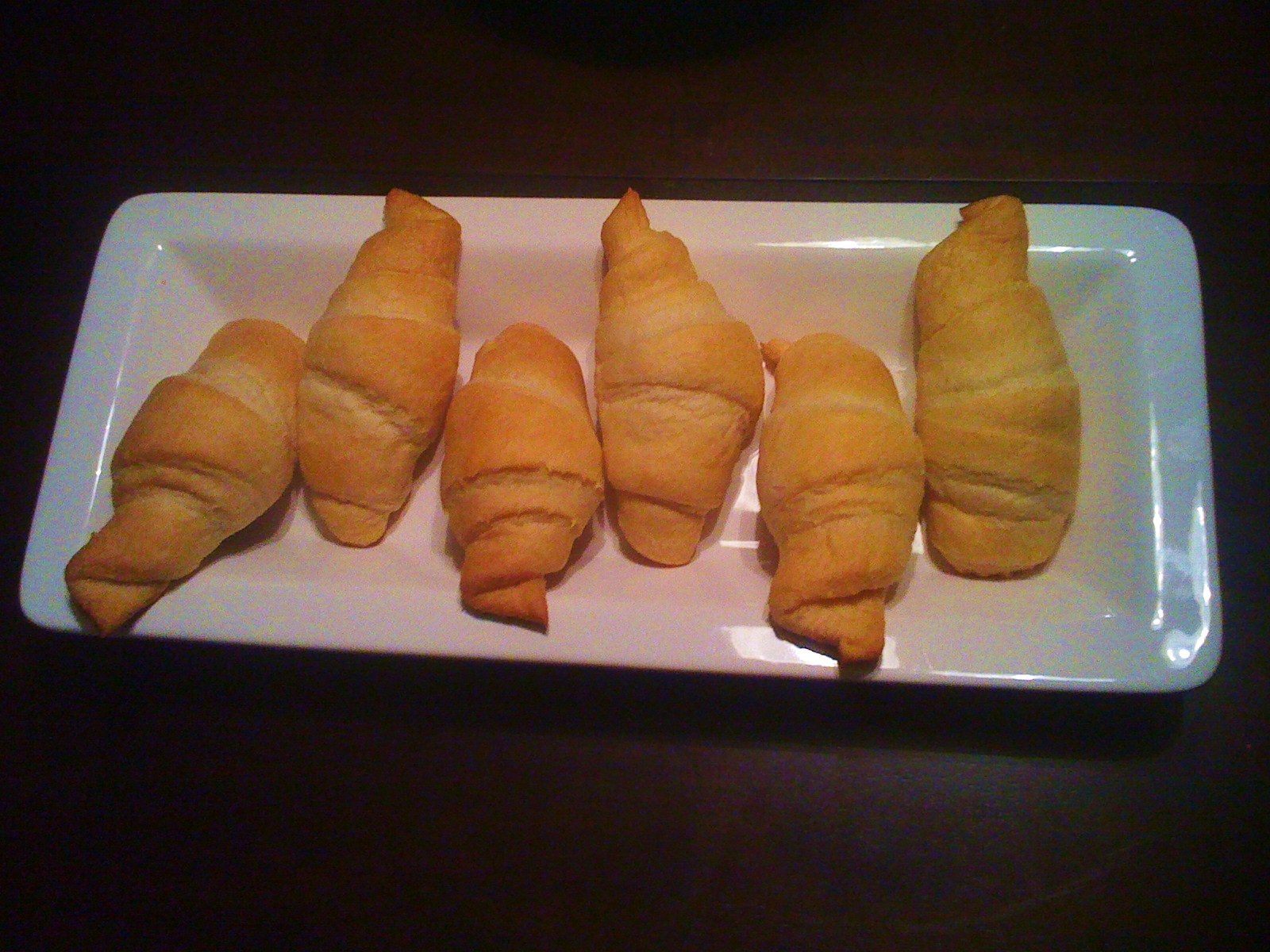The photograph features six golden brown, medium-sized crescent rolls that have been meticulously baked to an even, golden perfection. They are arranged in a staggered, side-by-side formation on a shiny, rectangular serving tray. The tray itself showcases a beautiful gradient of colors, shifting from light blue on the edges to an amber hue in the center. This elegant tray, which appears to be made of porcelain or a glassy coated metal, serves as a striking contrast to the solid black background of the image. The crescents exhibit the characteristic tapering at the ends and are thick in the middle, highlighting their well-wrapped, freshly baked nature. The entire arrangement sits atop a dark wooden table, adding to the composition's visual appeal.